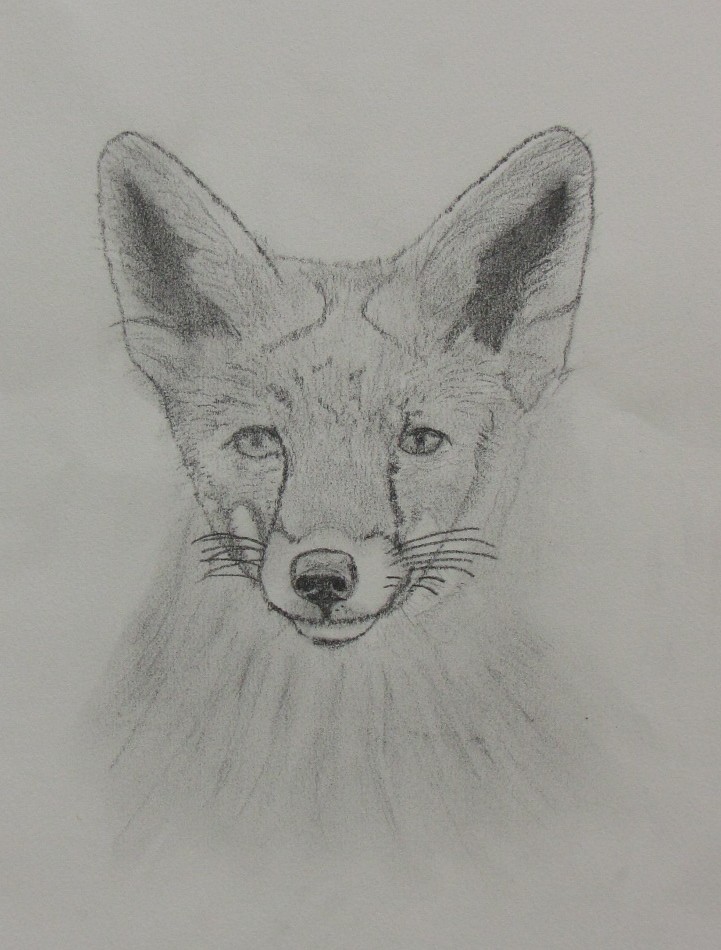This pencil drawing of a fox, created on a stark white sheet of paper, captures the front-facing visage and upper chest of the animal with intricate detail. The fox's large, pointed ears are prominently visible, and the shading within them suggests a depth and darkness that contrasts with the lighter, more delicate lines of the surrounding fur. The artist has employed thick lines down the fox’s nose, giving prominence to this central facial feature. The fur on the face is skillfully shaded in darker tones, highlighting the natural texture and contours, while the area around the muzzle remains unshaded, hinting at the white fur typically found in that region. Long, black whiskers extend outward from the fox's nose, adding to the realism. The neck and upper chest of the fox, though less detailed, are depicted with a combination of lines and shading, implying the texture and flow of the fur without overwhelming the viewer with detail. This meticulous portrayal effectively conveys the elegant and wild nature of the fox.